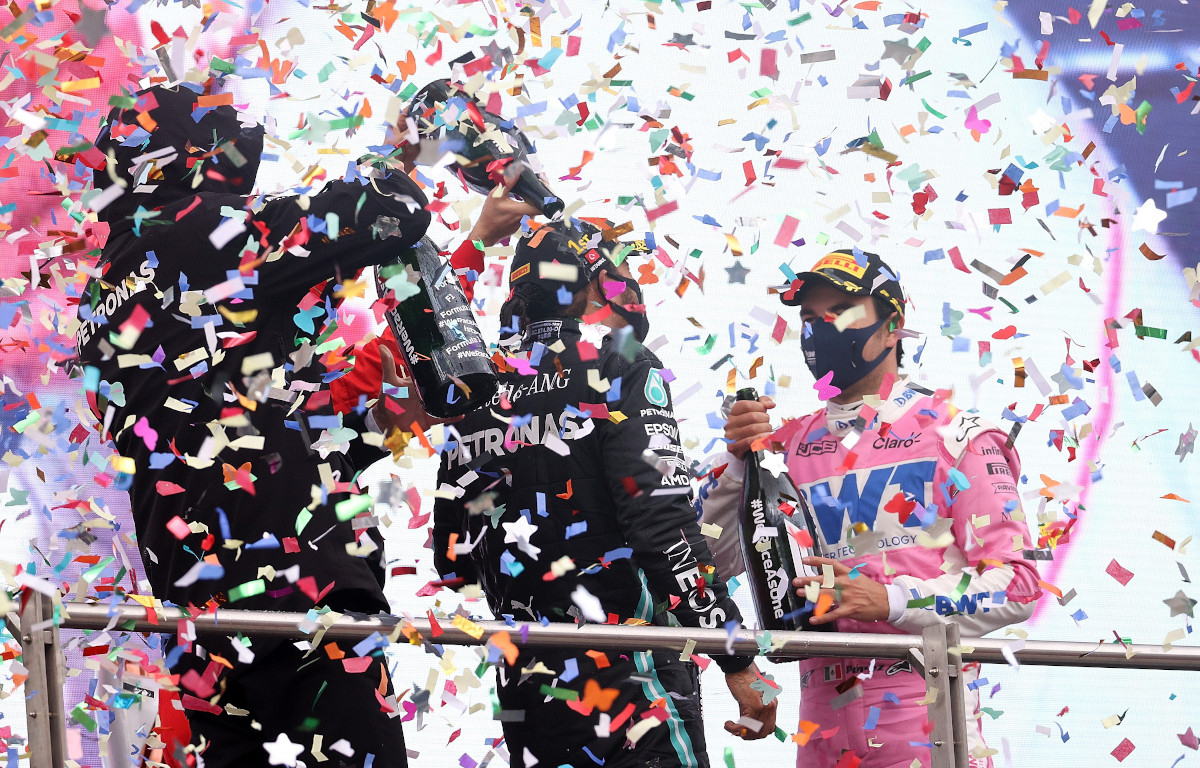The photograph captures a jubilant celebration following what appears to be a race victory. Dominated by a cascade of vibrant, multicolored confetti in pink, blue, white, and red, the image showcases three gentlemen on a stage. The central figure, dressed in a distinctive pink race suit emblazoned with the letters "WT" and wearing a face mask and cap, clutches a bottle of champagne triumphantly. Flanking him are two other racers in black suits, one enthusiastically pouring champagne over his fellow competitor. The scene is set against a background that features silver railings and a mix of colors, including a striking pink swirl and blue accents, all highlighting the raw elation and celebratory chaos of their victory moment.